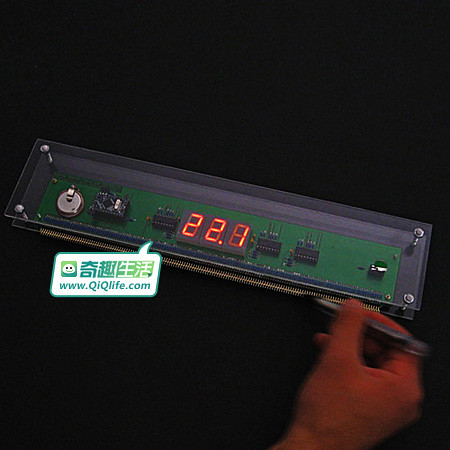The photograph is a color image featuring a stark black background devoid of texture, creating a one-dimensional, flat appearance. In the foreground, there is a human hand with a reddish tint, slightly blurred, possibly belonging to a man, with only a small part of the wrist visible. The hand holds a black ink pen, or possibly tweezers, and is positioned above a rectangular piece of equipment.

The equipment, appearing to be a tool for measuring or some kind of circuit board device, sits centrally in the image. The device has a gray casing with screws securing a clear glass or acrylic top, revealing a green circuit-like background underneath. Adorned on the equipment is a tag prominently displaying the web address "www.qiqlife.com" and features a small green smiley face icon along with symbols resembling another language. There is also a red digital display on the equipment showing the number 22.8. The detailed setup, with various protruding parts and components, suggests a meticulously designed electronic tool likely used indoors.